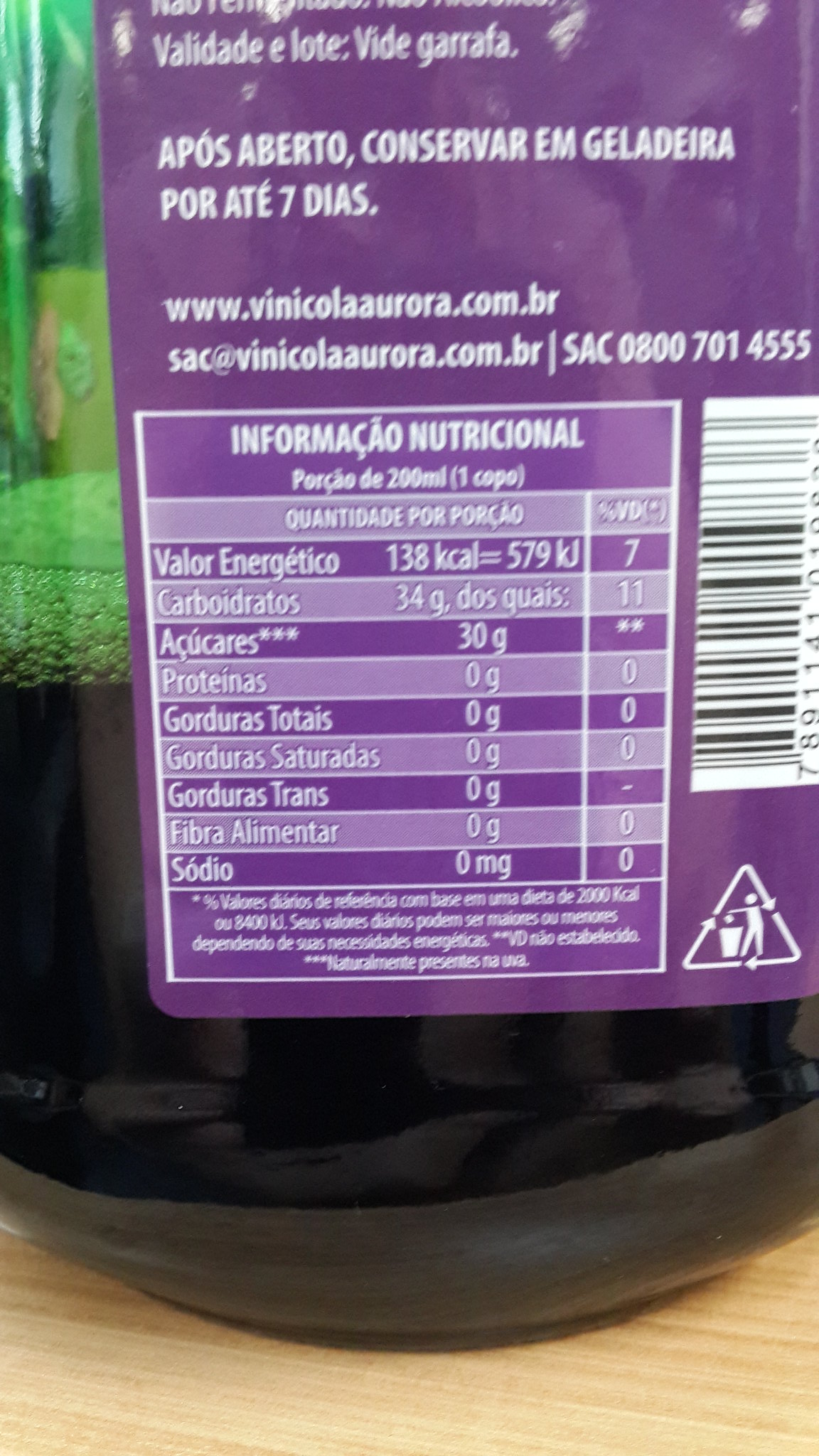The image features a green bottle with a purple label displaying nutritional information for a Spanish drink. The label text is entirely in white and includes details such as 138 calories per 200 milliliters serving. The drink inside the bottle appears to be a dark, foamy liquid, though most of it has already been consumed, leaving only an inch or two remaining at the bottom. The bottle sits atop a wooden table, and the glass's green hue is visible through the empty portion. Despite the linguistic barrier, the embellished label hints at the beverage's unique and possibly traditional origins.